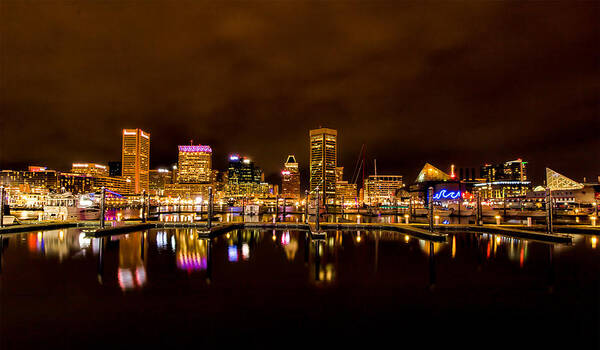This is a highly detailed night photograph of a vibrant city skyline taken from a dock. The image showcases a diverse array of brightly lit buildings, including several high-rises and angular structures, which are illuminated in an array of purple, blue, yellow, white, and orange hues. The skyline contrasts dramatically against a nearly black sky, with faint hints of gray clouds possibly due to moonlight. The water in the foreground is calm, reflecting the cityscape in a slightly blurry manner, adding an artistic element to the scene. The reflection in the water makes the image particularly interesting as it creates a mirrored, albeit imperfect, version of the skyline. In addition to the buildings, there are some smaller elements such as boats visible near the docks, reinforcing the bustling nature of this nocturnal urban landscape. The city lights not only illuminate the buildings but also create a vivid interplay of colors on the water, highlighting the city's active nightlife.